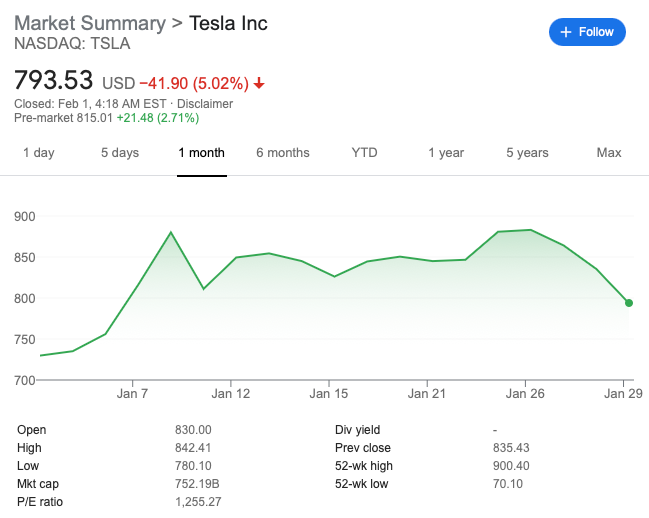This detailed caption is for an image of a stock price chart for Tesla Inc.:

---

The image displays a price chart for Tesla Inc. (ticker: TSLA) as provided by NASDAQ. In the top left corner, the title "Market Summary Tesla Inc." is visible. The chart shows a closing price of $793.53 as of 4 a.m. Eastern on February 1st. This price is highlighted in red, indicating a decrease of $41.90 or 5%.

The chart shown is configured to display the stock's performance over a one-month period, from January 7th through January 29th, with price variations ranging between $700 and $900. The price trend is depicted by a green line which initially rises slightly from January 7th, approaching but not reaching $900. The line then experiences a dip before January 12th and fluctuates moderately until a significant drop is seen on January 29th at $793.53.

At the bottom of the graph, key metrics are listed: 
- Open: $830.00
- High: $842.41
- Low: $780.10
- Market Cap: $752.19 billion
- PE Ratio: 1,255.27
- Dividend Yield: Not provided
- Previous Close: $835.43
- 52-week High: $900.40
- 52-week Low: $70.10